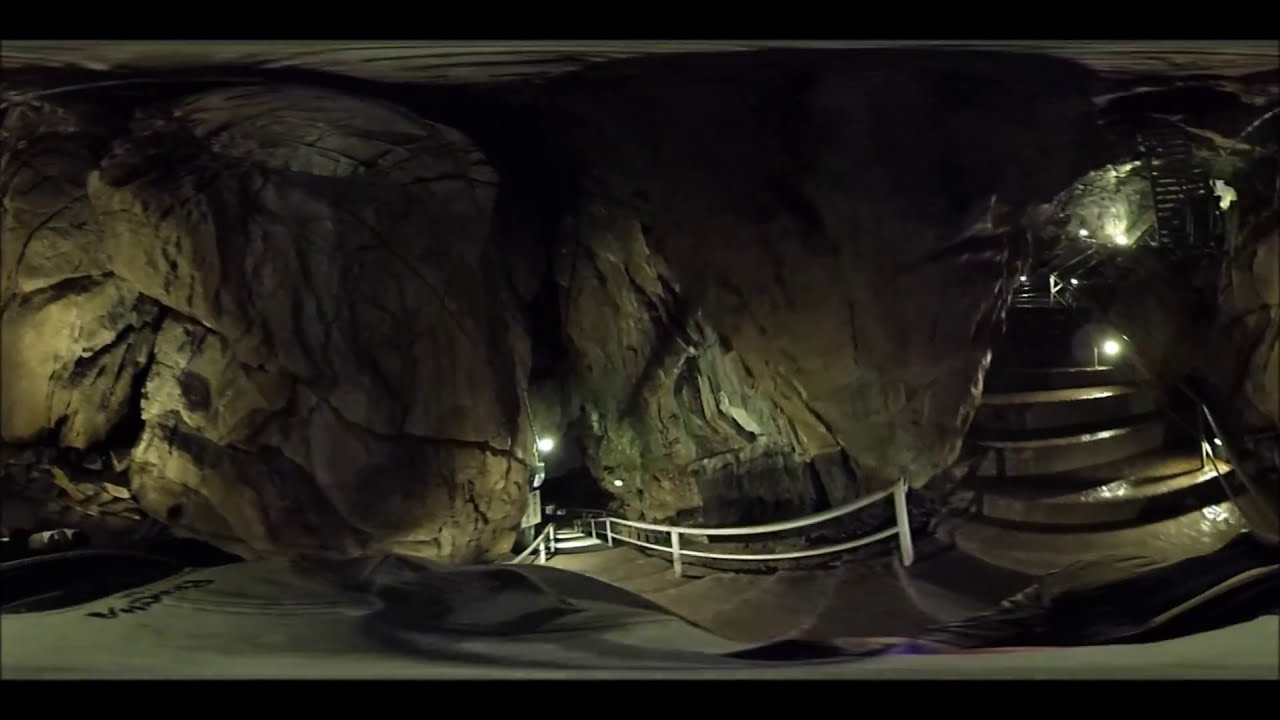This photograph captures the vast interior of a cavern in a wide-angle, landscape orientation with a fisheye-like distortion. The walls of the cave are made of irregular, jagged stone, displaying a variation of browns and grays with numerous cracks and chiseled textures. In the center of the image, a prominent man-made stairway descends, characterized by brown steps and white metallic railings on each side. The steps curve upward towards the right, leading into the upper sections of the cave. The cavern is illuminated by artificial lights installed on the ceiling, casting bright white light onto the scene, although certain areas remain shrouded in darkness.

On the right side, near the beginning of the stairway, there's a large metal structure resembling a warrior-style or Darth Vader-like helmet, stacked atop a metal base. This enigmatic object adds a unique focal point to the composition. Additionally, the photograph includes thin black bars at the top and bottom, potentially indicating framing or further distortion. A sign is visible, possibly providing information about the cave, enhancing the sense of depth and exploration within this remarkable underground space.